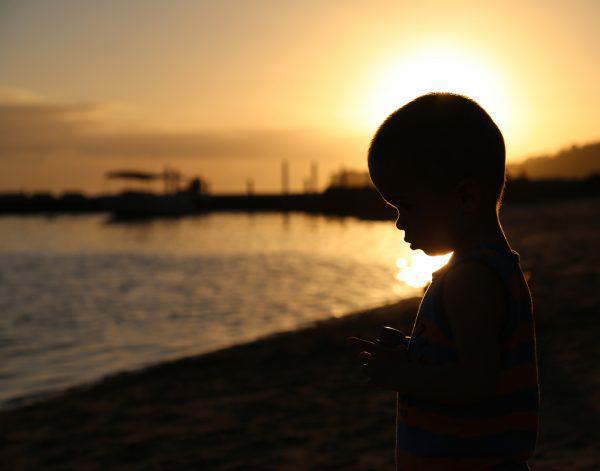The photograph, taken at either dusk or dawn along a shoreline, captures a poignant and moody scene. In the foreground, a child stands alone as a silhouette against the setting sun, their head bowed as if in contemplation or prayer. The child appears to be bald and may be wearing a sleeveless tank top. Their profile is the focus, with no discernible facial features due to the backlighting. The background features gentle ripples on the water, a distant dock, and boats scattered across the horizon. A tiny hill and some clouds can be seen in the distance, adding depth to the serene yet evocative landscape. The overall composition highlights the stark contrast between the child's dark silhouette and the radiant hues of the sunset, creating a powerful, emotive image.